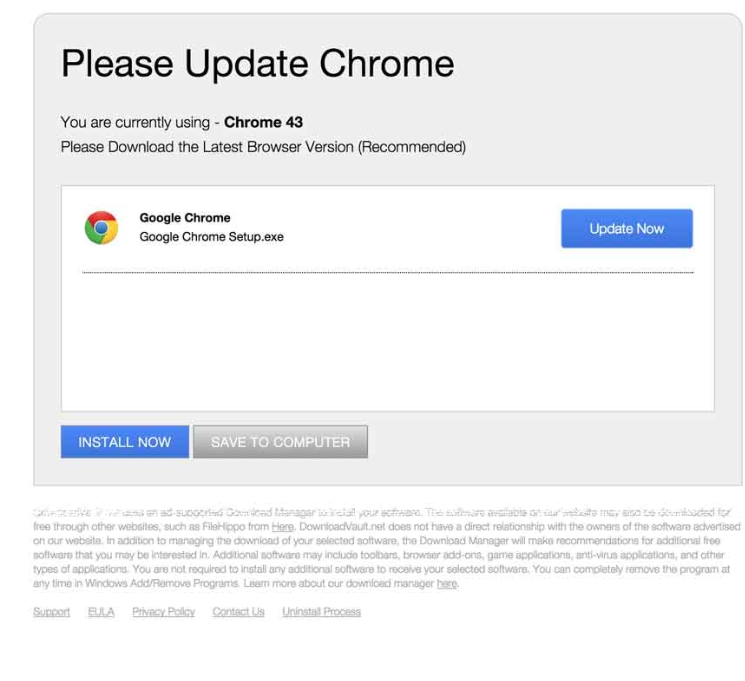This is a screenshot of the Google Chrome Update page prompting the user to update their browser. The background of the image is predominantly gray, providing contrast for the central white section. 

At the top left corner of this white section, located approximately one space from the top and left edges, there is a prominent message in large, bold font reading: "Please update Chrome." The words "Please," "update," and "Chrome" are all capitalized at the beginning.

Directly beneath this heading, in a smaller font, the message states: "You are currently using - Chrome 43," with "Chrome 43" displayed in bold to emphasize the version number.

Below this, there is a suggestion in smaller text: "Please download the latest browser version (recommended)."

Further down in the white box, the header "Google Chrome" appears, followed by the text "Google Chrome setup.exe." On the right side of this section, there is a button labeled "Update Now," providing a clear call to action for the user to proceed with the browser update.